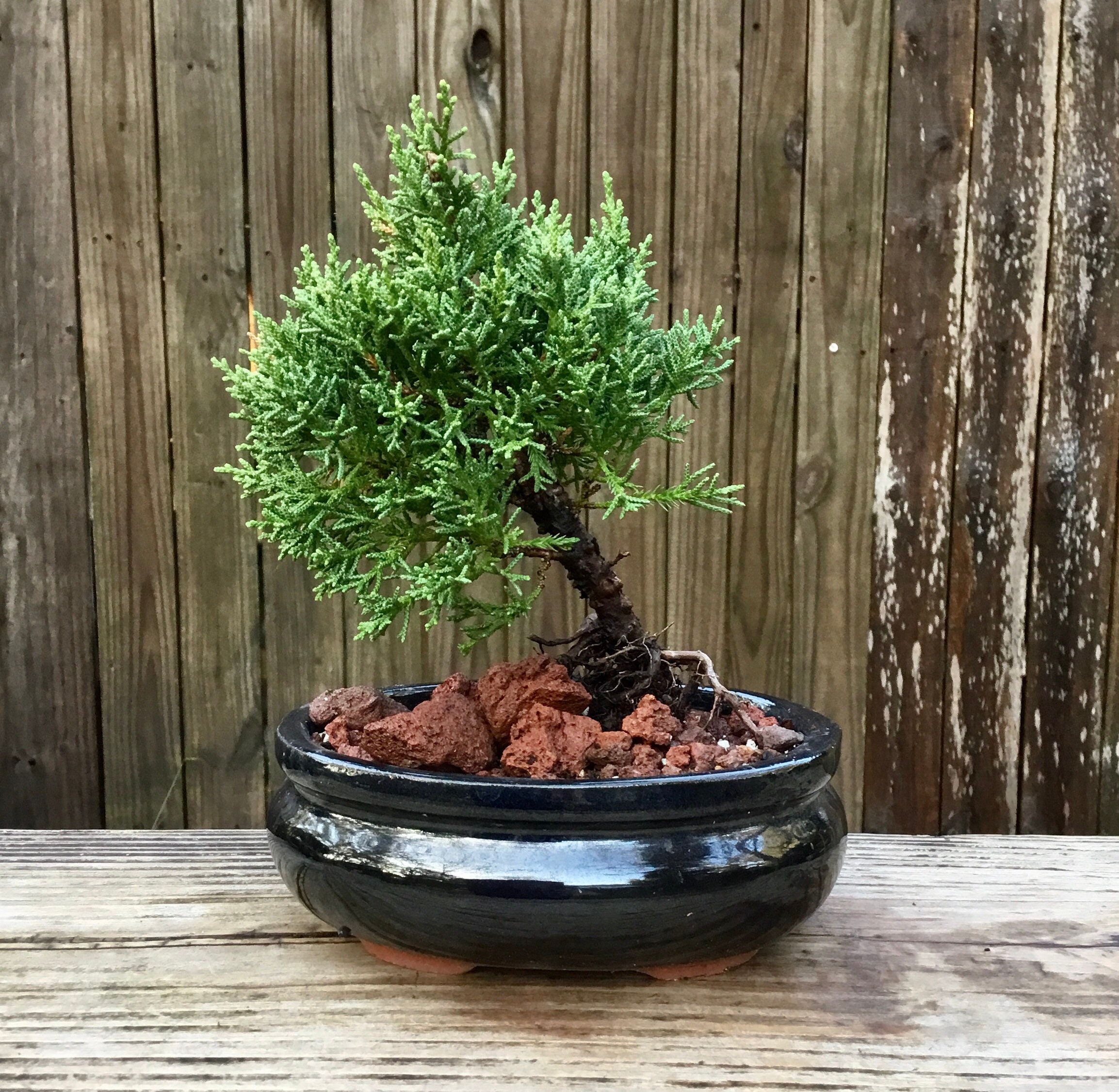The image depicts a vivid and detailed color photograph of a small bonsai tree, possibly an evergreen or pine, planted in a glossy black, shallow ceramic pot. The pot features red, terracotta-like rocks and visible roots. The bonsai, with its dark brown trunk, leans diagonally from the bottom right to the upper left. The tree boasts healthy, needle-like, dark green foliage. This arrangement rests on what appears to be a pale, weathered wooden table or shelf, which could be oak, placed outdoors. In the background, there is a fence made of vertical, weathered wooden boards, exhibiting various shades of gray and dark brown with some white speckles. The scene is brightly lit by natural sunlight, enhancing the vibrant green of the bonsai and casting reflections on the pot's glossy surface.